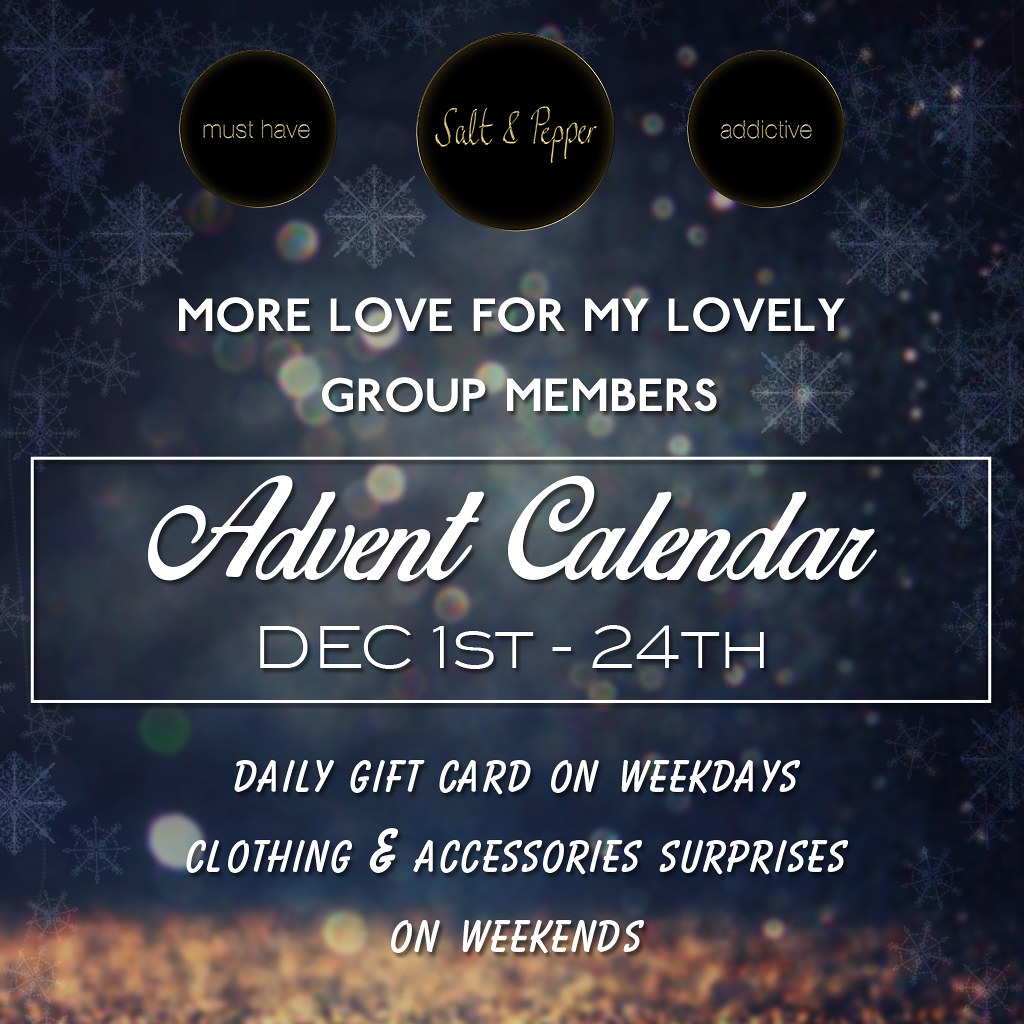This promotional poster, almost square in shape, features a festive blue wintry background adorned with snowflake patterns, giving it a Christmas feel. At the top, there are three gold-rimmed circles with the following text inside: "Must Have," "Salt and Pepper," and "Addictive." Below these circles, in white script, it reads: "More love for my lovely group members." Further down, it details an Advent Calendar running from December 1st to 24th, promising daily gift cards on weekdays and clothing and accessories surprises on weekends. The base of the poster transitions into a reddish-brown pattern that resembles autumn leaves, contrasting with the otherwise blue and wintry theme.